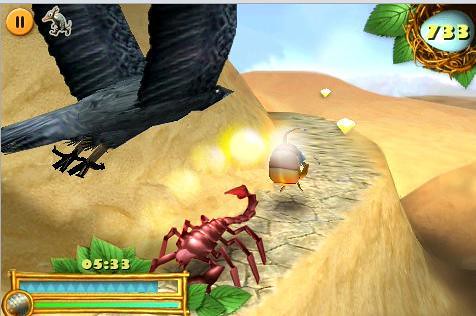In a vibrant scene from a video game, a rat-like creature is seen navigating a pathway. Dominating the center of the image is a large circular emblem displaying the number "733," from which numerous branches spiral out, adorned with leaves on both the left and right sides. The foreground features a mound of sand beneath a clear blue sky. Accompanying the pathway, a menacing scorpion with six legs, two arms, and a pincer prowls nearby. The bottom left corner of the image shows a nearly filled blue bar labeled "05.133," beneath which lies a green bar. On the far right, the sandy terrain slopes downward, framing the dynamic scene.